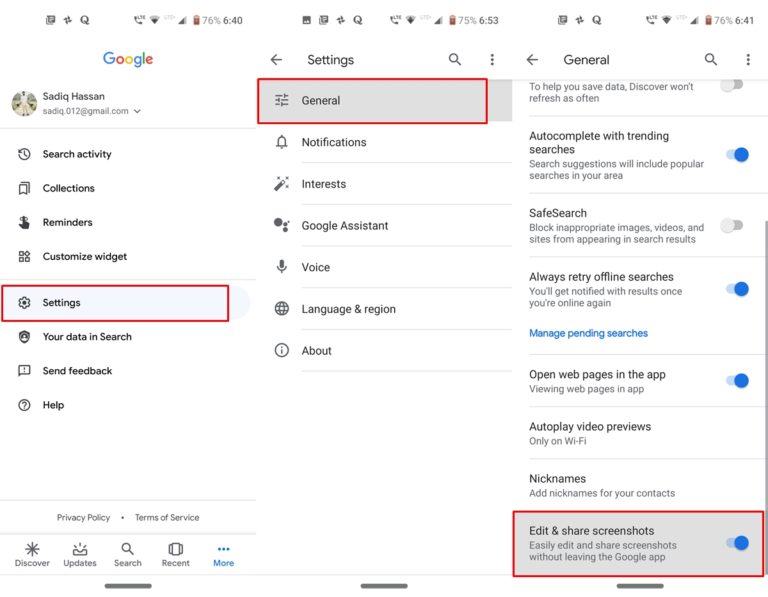In this composite image, we observe three screenshots showcasing various details on a smartphone. 

- **Left Screenshot**: The time displayed is 6:40, and the battery percentage is at 76%. 
- **Middle Screenshot**: The time shows 6:53, with the battery slightly decreased to 75%. 
- **Right Screenshot**: The time here reads 6:41, with the battery percentage again at 76%. 

Despite the time differences, the screenshots share identical icons and interface elements. Visible icons include Messages, Photo App, Quora, LTE, Wi-Fi signal, and network signal bars. Various menu text items are also present, including but not limited to General, Notifications, Interests, Google Assistant, Voice, Language (Norwegian), and About.

Additionally, to the left side of the image, user-specific information is detailed:
- **User**: SARDIC Horizon
- **Username and Email**: sardic012@gmail.com
- **Options Visible**: Search activity, Collections, Reminders, Settings, Your data in search, Send feedback, Help
- **Settings Status**:
  - Auto-complete with trending searches: On
  - Safe search: Disabled
  - Edit and share screenshots: Enabled

This carefully assembled image offers a snapshot of the user's digital environment, highlighting differences in time and battery percentage while maintaining consistent visual and textual elements across the interface.